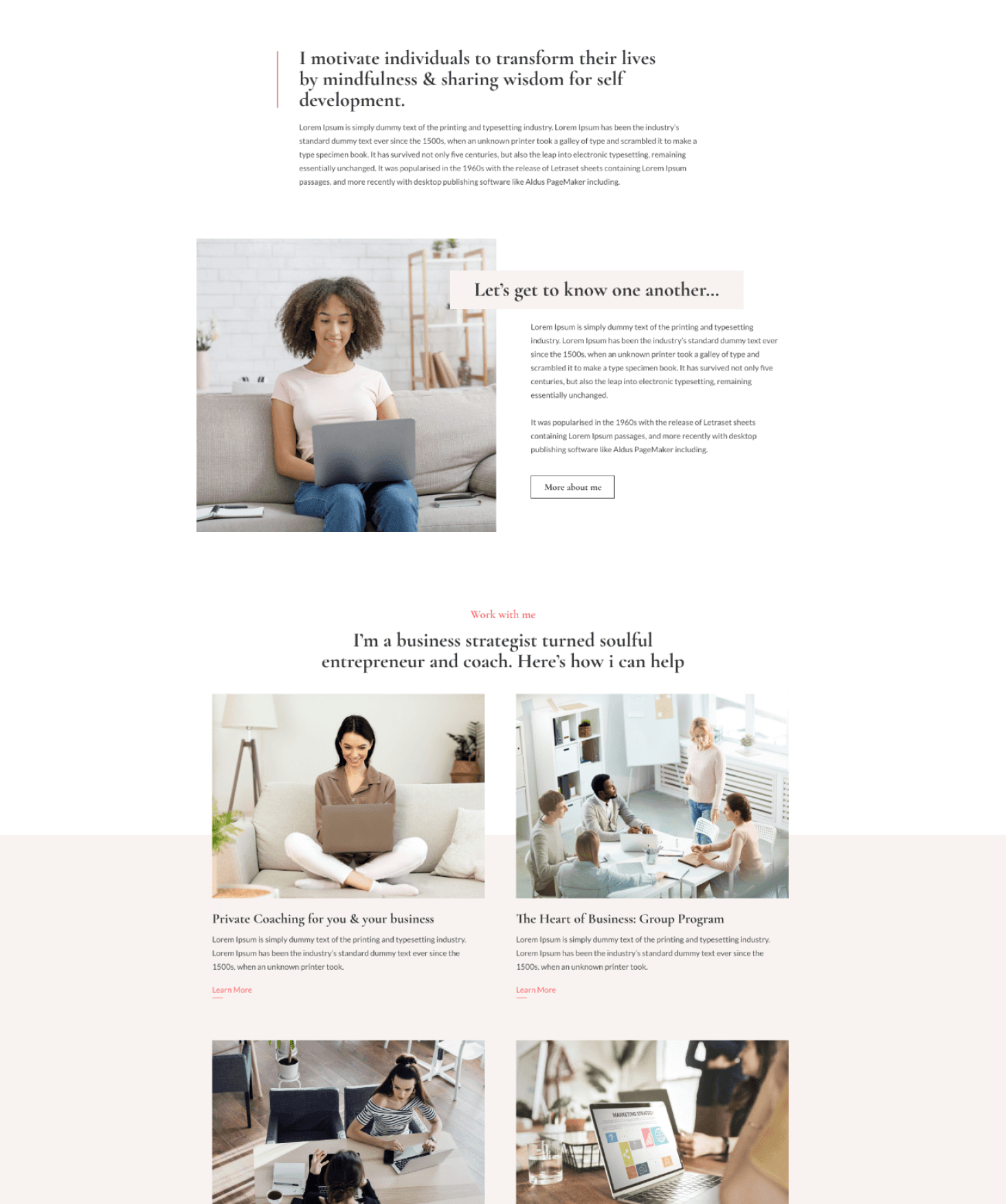This advertisement screenshot showcases a tranquil and inviting promotional layout for a mindfulness and self-development program. At the top, a headline proclaims, "I motivate individuals to transform their lives by mindfulness and sharing wisdom for self-development," setting the tone for the offerings described. Beneath this, a paragraph elaborates on the approach and benefits of the program.

Central to the screenshot is an image of a woman seated on a couch, engaged with a laptop. The text overlay reads, "Let's get to know one another," accompanied by another paragraph detailing the services. A clickable button invites users to explore further, underscored by the woman's professional introduction: "I'm a business strategist turned soulful entrepreneur and coach. Here's how I can help."

Adjacent to this, the advertisement highlights four smaller images depicting various group settings. These images emphasize the diversity of the program offerings, including group programs and one-on-one coaching sessions. The serene and cohesive aesthetic, characterized by light peach tones and calming colors, enhances the zen-like atmosphere. The photographs feature real people in genuine settings, contributing to the authenticity and relatability of the advertisement. Even the attire of the individuals is thoughtfully chosen to maintain the overall calm and collected aesthetic.